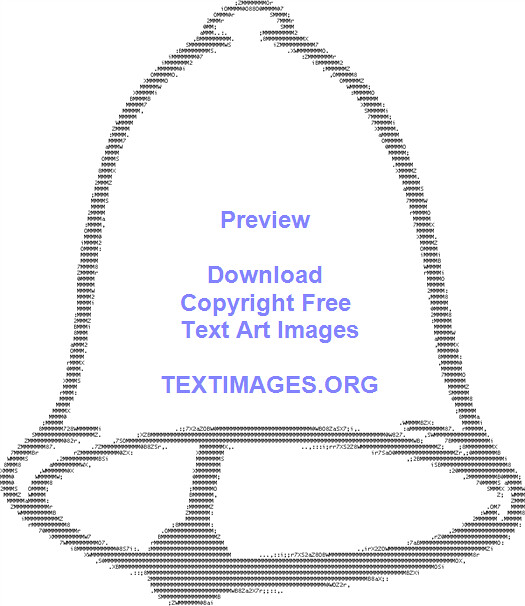This is a digitally created text image of a bell, characterized by a striking black and gray outline, which is composed of pixelated lines arranged horizontally. The interior of the bell is completely white, creating a stark contrast against its detailed outline. This outline is intricately formed using characters from the ASCII table, predominantly M's and heart shapes, which contribute to a thick and defined appearance. The bell features a knob at the top, gracefully curving down to a rounded bottom where a clapper is depicted swinging to the left. In the center of this bell-shaped text image, written in prominently a purple and blue hue, is the text "Preview, download copyright-free text art images, textimages.org." The website name "textimages.org" is capitalized, while the rest of the text follows standard capitalization rules, enhancing its readability and aesthetic appeal.